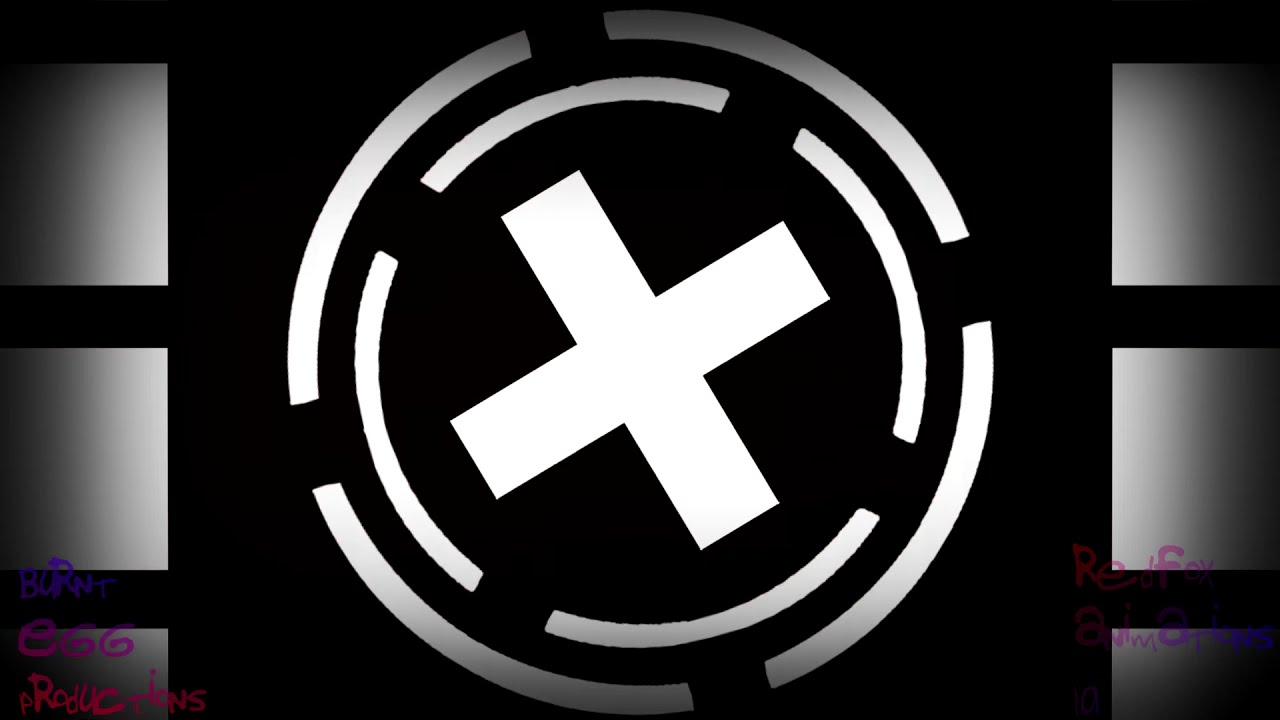The image appears to be a digitally created artistic picture dominated by shades of black, gray, white, purple, pink, and off-reddish-orange. On the outer left and right sides, there are three gray squares set against a black background, with the bottom square cut off. The central section of the image features a large black square enclosing two concentric white circles with four breaks in each, creating an off-center alignment. At the very center, a slightly tilted equilateral cross or plus sign, resembling a large white "X," is prominently displayed. In the lower left-hand corner, text reads "Burnt" in purple letters, followed by "E66" in pink, and "Productions" in a hot pink or off-reddish-orange shade. Similarly colored text appears in the lower right-hand corner, but it is too faded to be legible. This image likely represents a company logo or might be used in a presentation setting.